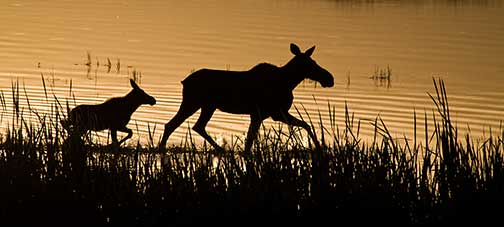The image is a color photograph in landscape orientation, capturing the silhouette of two animals, likely a moose and its young calf, walking in profile from left to right. The larger adult moose is positioned prominently in the center with the smaller calf slightly behind it. Both faces are turned towards the right, with their back legs extending toward the left side of the image. The top 60% of the background is filled with water, which is reflecting a warm orange hue from the setting sun, creating a serene and picturesque scene. The water shows subtle ripples and a few sporadic stalks of grass protruding from it. The bottom 40% of the image showcases the land, which is a dark silhouette teeming with various blades of tall grass. This distinct division of water and land frames the moose and calf, emphasizing their forms in a striking photographic representational realism style.